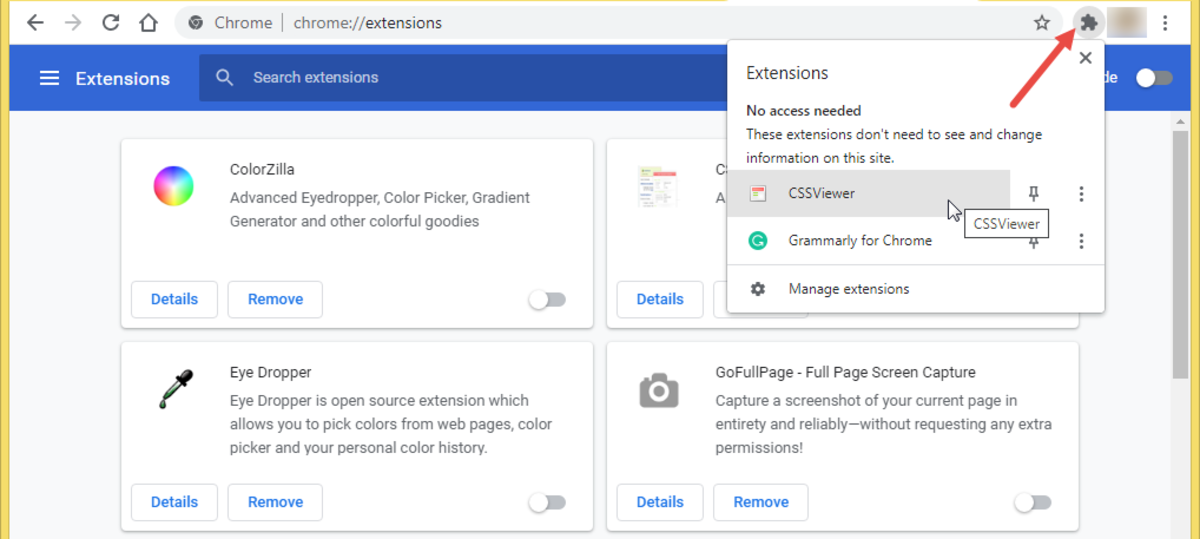A detailed and cleaned-up caption for the image described would be:

"The screenshot displays the Extensions page on Google Chrome, with a focus on a drop-down menu for managing browser extensions. In the upper right-hand corner, the gray puzzle piece icon represents the Extensions on Chrome, highlighted by a red arrow pointing towards it. A drop-down menu labeled 'No access needed' informs that the listed extensions do not need access to view or change information on the current site. The CSS Viewer extension is highlighted, indicated by the mouse cursor hovering over it. To the right of CSS Viewer, there is a pin button. Below it, the Grammarly for Chrome extension is listed, also accompanied by a pin button next to it and a cog wheel icon labeled 'Manage Extensions' below that.

At the top of the page, the address bar shows 'chrome://extensions'. The blue header features a three-bar icon for additional options on the left, the word 'Extensions' in white, and a darker blue search bar labeled 'Search Extensions'. Below the header, a list of additional extensions includes ColorZilla, Eyedropper, and GoFullPage - Full Page Screen Capture."